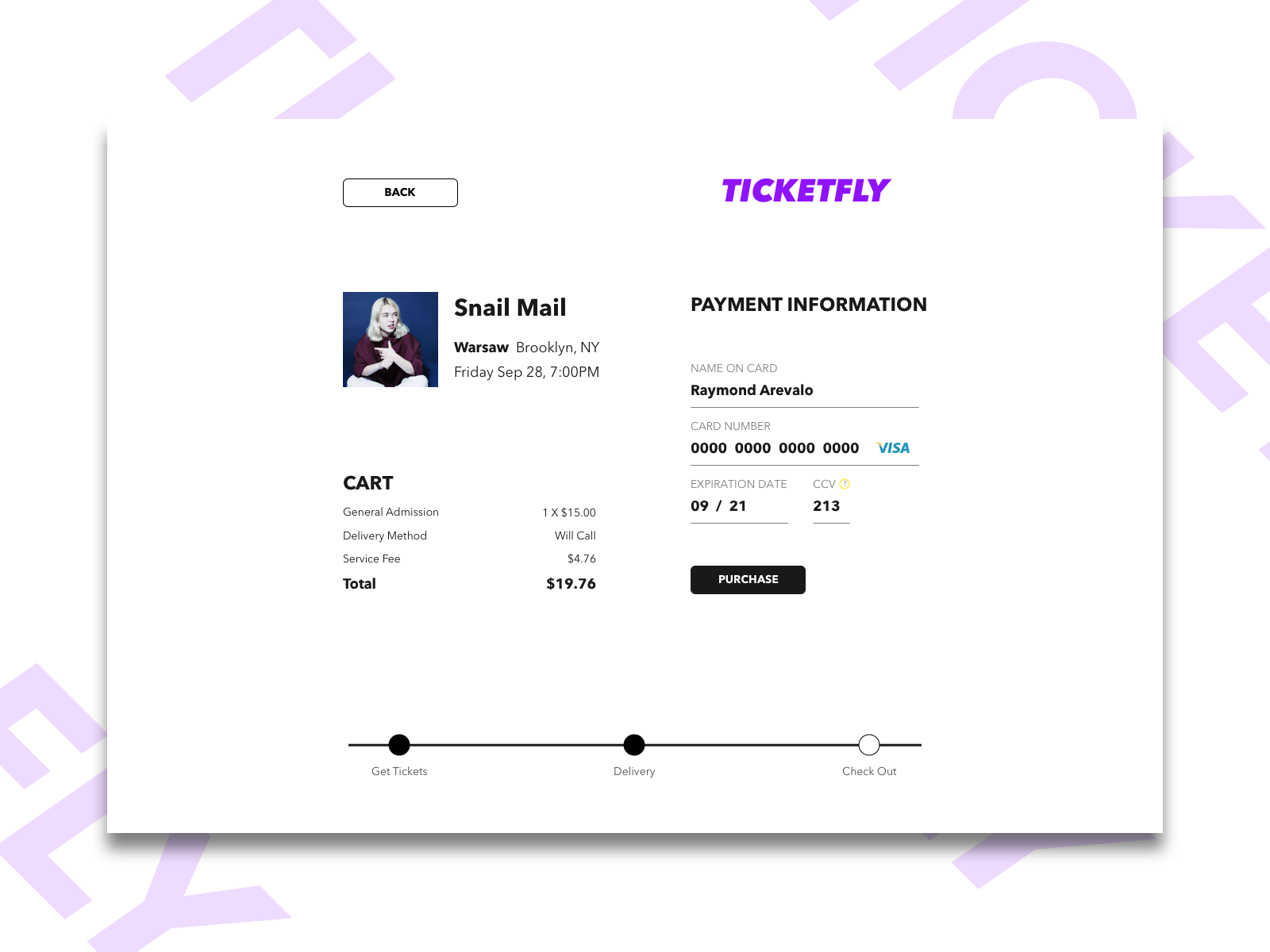A screenshot from a website showing the purchase checkout page for an event ticket. The page is superimposed over a white background, featuring diagonal, large purple text partially visible with letters "F-L-Y" appearing in the bottom left-hand corner, and other fragments like “T-I” in the upper left and “I-C-K-E” in the upper right, partially obscured by the page. The page has a shadow underneath it, creating a three-dimensional effect.

In the upper left-hand corner, a “Back” button is displayed along with details for an event: "Snail Mail," "Warsaw," "Brooklyn, NY," set for Friday, September 28th at 7 PM. To the left, there is a picture of a woman with blonde hair, wearing a red top and white trousers, sitting with her arms together against a blue background.

Underneath the image is a section titled "CART," where the ticket details are listed: "General Admission: $15," "Delivery Method: Will Call," "Service Fee: $4.76," totaling $19.76. "Ticketfly" is written in purple in the upper right corner of this section.

Further down, payment information fields are displayed, with the name on the card shown as "Raymond Arvarello," a card number represented by a series of zeros, marked as a Visa card, with an expiration date of "09/21" and CCV "213." Below this, there is a black "Purchase" button with white writing.

At the bottom of the page, a horizontal black line with some circles contains three steps: "Get Tickets" with a filled black circle, "Delivery" with a filled black circle, and "Check Out" with an empty white circle, indicating the current step in the checkout process.